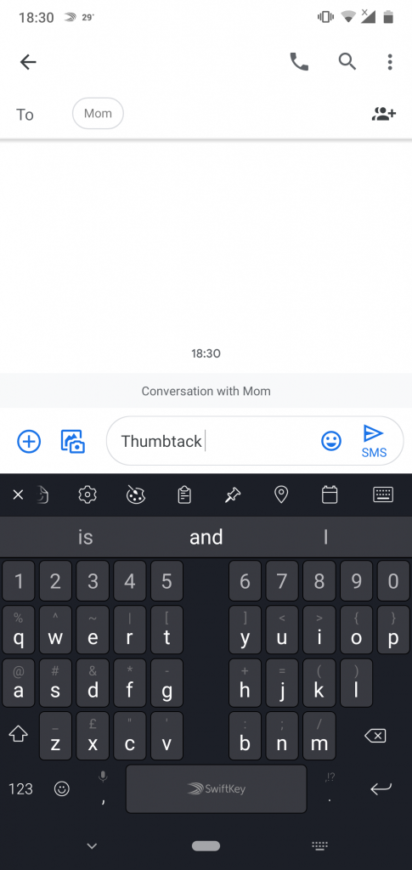This is a screenshot of a mobile device displaying a text messaging app. The recipient at the top of the screen is labeled as "Mom." The conversation thread itself is currently empty, with a completely blank, white background. In the keyboard input field, the user has started typing the word "thumbtack." The keyboard is displayed in a sleek black theme, with white letters on the keys. Autocorrect functionality is active, offering typing suggestions. To the right of the input field is an icon that allows the user to attach a picture to the text message.